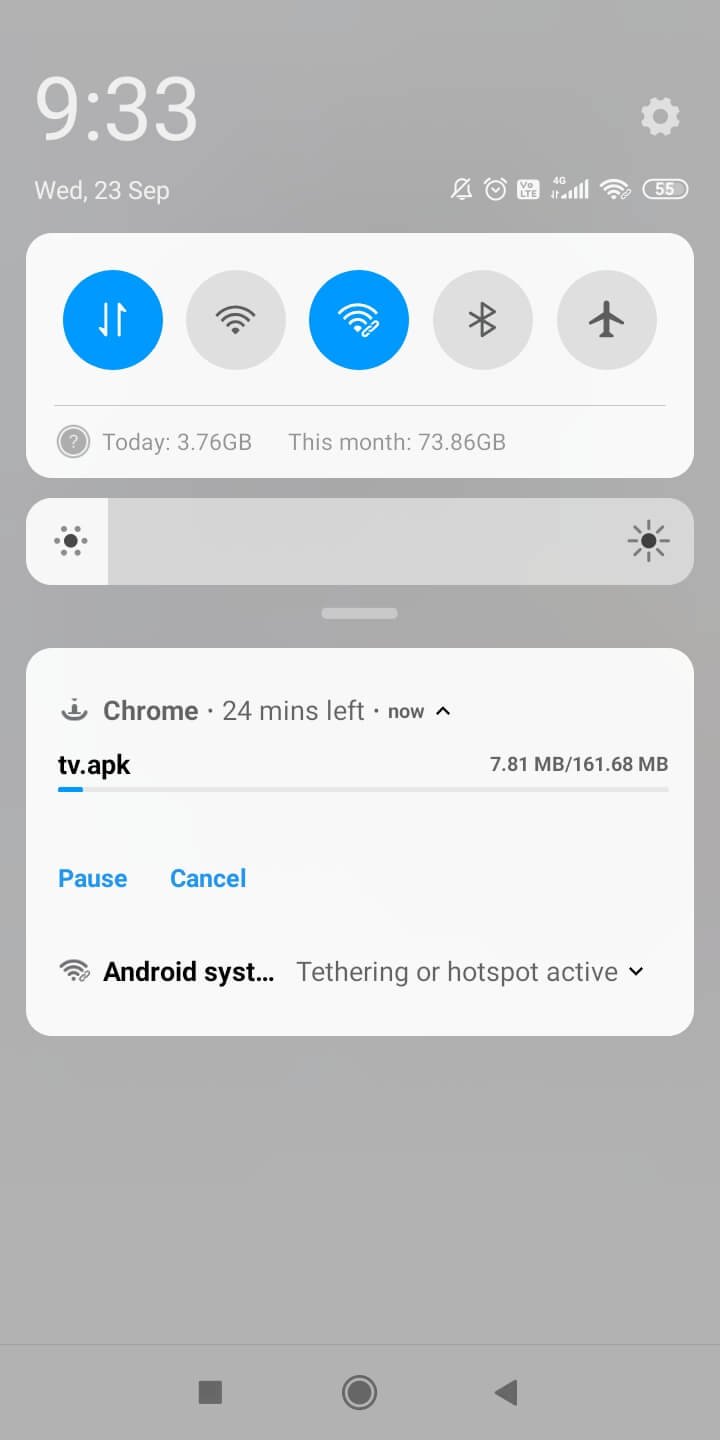This image is a screenshot set against a light gray background, depicting a smartphone interface. In the upper left corner, large bold text displays the time as "9:33." The upper right corner features a white settings icon. Directly beneath the time on the left, the text reads "Wednesday 23rd September." To the right of this date information, there are white icons indicating notifications, an alarm clock, and an LTE connection. The Wi-Fi is shown as being active, and the battery icon displays a small number "55," indicating the battery percentage.

Below this section is a white rectangular box displaying round buttons for Wi-Fi, Bluetooth, and Airplane mode. Underneath this, in gray text, it reads "Today 3.76 GB, This Month 73.86 GB," likely indicating data usage statistics.

Further down, another white box appears with gray text in the upper left corner stating, "Chrome 24 mins left." An upward-pointing arrow accompanied by the word "Now" suggests an ongoing action. Within this box, a blue progress line on a horizontal gray bar indicates that a file named "tv.apk" is currently downloading. At the bottom of this image, a message in gray text reads, "Thank you for watching."